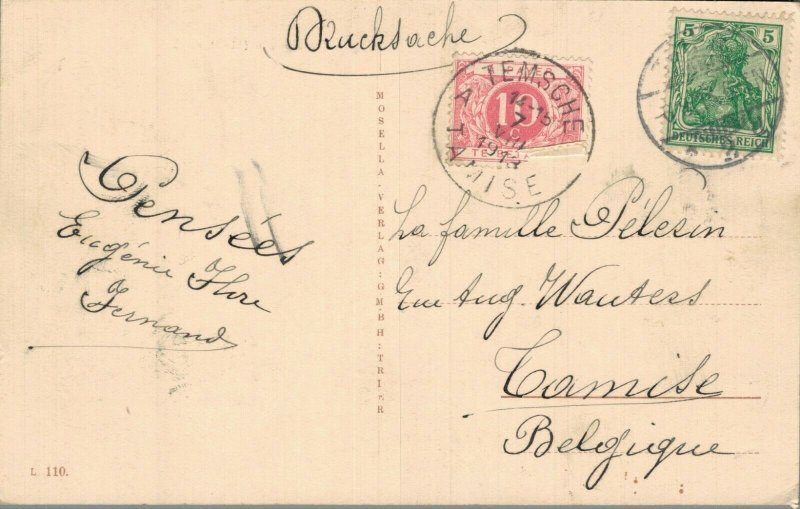The image showcases a vintage postcard, evident from its worn and slightly faded appearance, suggesting it dates back to the year 1913. The postcard, predominantly in a light pinkish hue, bears elegantly penned cursive script in a language other than English. The address on the postcard reads "La Famille Helensen," indicating it might be intended for a family in Belgium, as it mentions "CAMISE BELGIQUE" as part of the address.

In the top right corner, there are two distinct stamps. One is a reddish-pink square stamp with the number 10, partially obscured by a black postmark resembling a form of approval. Adjacent to it is a greenish stamp that bears the inscription "Deutsches Reich" and the number 5 in the upper right corner, also marked by a postmark with the word "T-E-M-S-C-H-E” encircling it.

The postcard's surface is covered in neat cursive writing, though challenging to read, featuring both at the top and along four lines in the main body, with an additional three lines on the right side. The combination of the elegant script and the foreign language gives the postcard a further sense of antiquity and historical mystique.